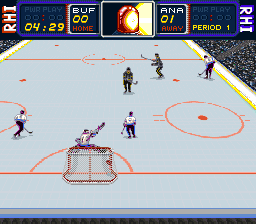This is a small, square image capturing an eight-bit hockey video game, likely on the SNES (Super Nintendo Entertainment System). At the top of the screen, there's a prominent scoreboard banner. On the left side of the banner, it displays "Buff" for Buffalo, showing a score of 0-0, indicating they are the home team. Adjacent to this, there's a small, unhighlighted blue square labeled "Power Play 00-00." The time remaining, highlighted below, reads 4:29. Centrally located within the banner is a box featuring a siren icon. On the right side, it reads "Anna" for Anaheim, with a score of 1, marking them as the away team. Above this, the Power Play status again reads with zeros, and at the bottom, it confirms the game is in "Period 1" with yellow text.

The game's main action is happening near a goal on the ice rink. The goal, featuring red piping, is situated slightly left of center. A goalie is positioned directly in front of the net, performing a split with one arm extended to the upper right. Two defensive players in white jerseys support the goalie near the net, one skating to the left and the other standing to the right. Additional players can be seen in the background, with two in black jerseys—the away team's colors—moving towards the goal. This vividly detailed scene captures the dynamic moment of play in this nostalgic hockey game.